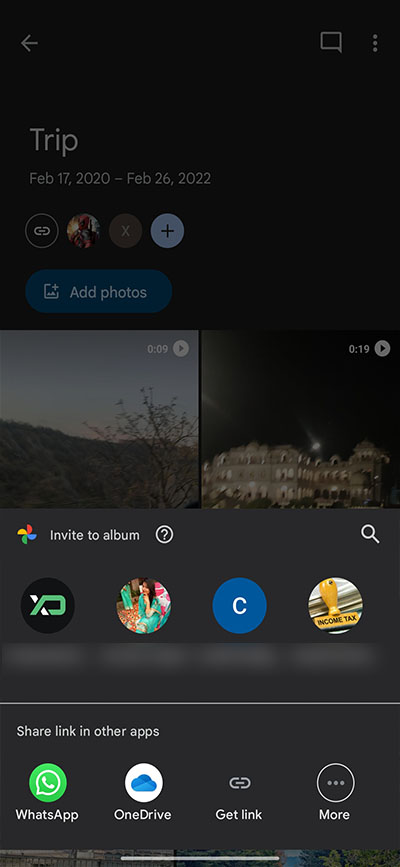In this image, a pop-up menu is displayed on the bottom half of the screen, activated by clicking the share button. The pop-up menu has a slightly grey background and prominently features the text "Invite to Album" in white, positioned on the top left. Next to this text is a colorful icon of a Google Photos fan, featuring green, yellow, red, and blue segments. Adjacent to the text is a small question mark icon. 

On the right side of the pop-up, there's a search icon represented by a magnifying glass. Below, four user profiles are visible: the first is marked with "XD" in black, green, and white; the second profile features a woman's image; the third profile is marked with a blue "C"; and the last profile on the right is labeled "Income Text." At the bottom of the pop-up, there are options for sharing: "Share link in other apps," with icons for WhatsApp (green and white), OneDrive (white and blue), "Get link" with a link icon, and "More" represented by an ellipsis button.

The upper portion of the image, which is the main application page from which the pop-up originates, identifies the album titled "Trip February 17, 2020, to February 26, 2022." It prompts the user to "Add photos,” and shows that two videos have been selected for sharing. The background is black, indicating it is within the Google Photos app. The first video, located towards the left center, has a duration of 9 seconds, while the second video on the right has a duration of 19 seconds.